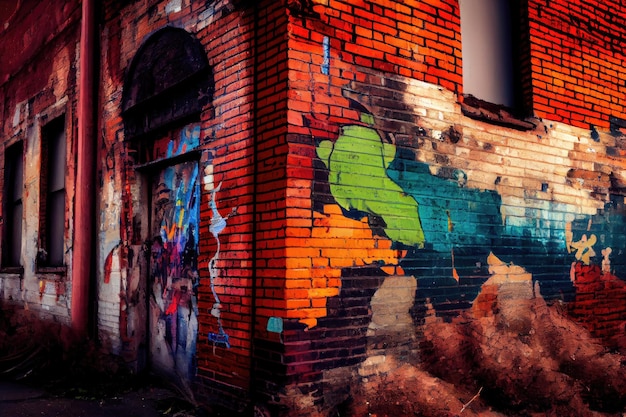This image features an abandoned, red brick building prominently viewed from the corner, highlighting its two converging walls. The building exhibits a mix of vibrant, abstract graffiti art. The left wall displays two windows and a door with a dark archway, adorned with an array of colorful paint—blues, yellows, oranges, and reds—reflecting a sense of decay and artistic expression. The right side features another window alongside more graffiti, including green and blue shapes that resemble clouds or undefined forms. The detailed red bricks are contrasted with gray grout, giving the façade a distressed look. A notable pipe runs along the building's exterior, matching the brick's hues, while a white blank spot or window space adds to the dilapidated appearance. The photograph, likely taken during late hours with dim lighting, uses filters to accentuate the colors, enhancing the surreal, almost night-time ambiance of this derelict yet art-covered building. A sidewalk in front of the building completes the scene, emphasizing its urban context.